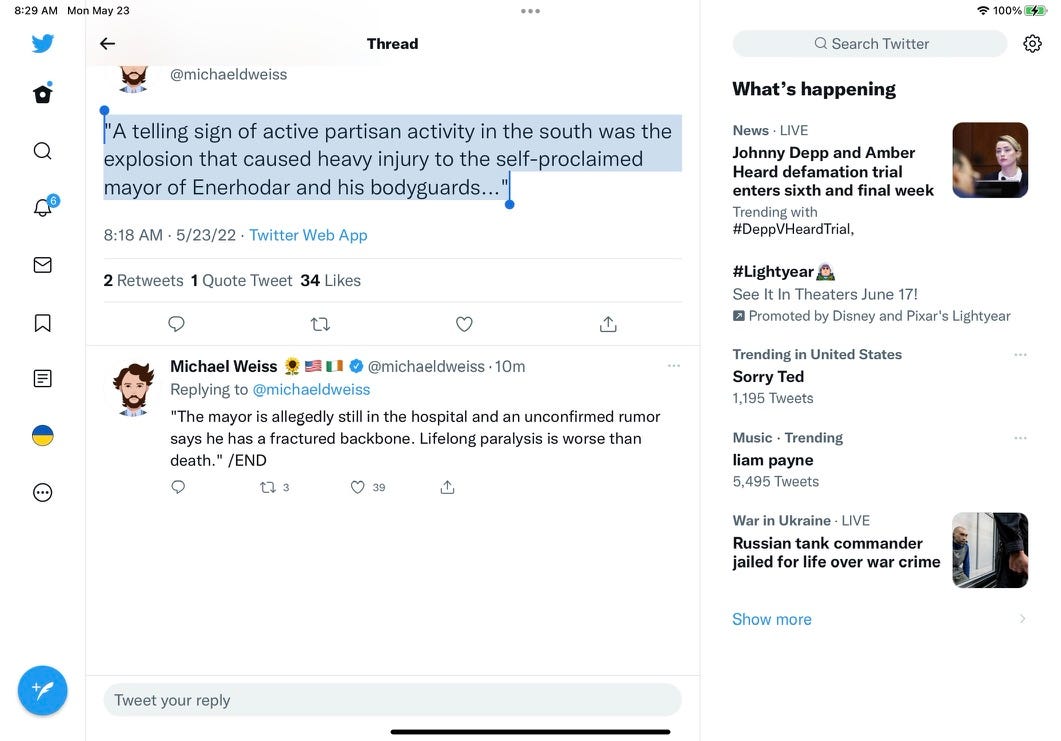A detailed caption for the described image:

"An open Twitter webpage is displayed on a desktop monitor, showcasing the platform's classic three-pane layout. The left pane contains fundamental navigation links including Home, Search, Notifications, Bookmarks, and other standard options. The central pane is the main feed where tweets are visible. Two tweets from an individual named Michael D. Weiss are prominently featured. In his first tweet, Michael discusses the implications of partisan conflicts in the South, highlighting an explosion that severely injured the self-proclaimed mayor of Enerhodar and his bodyguards. The tweet details that the mayor is still hospitalized, with unconfirmed rumors suggesting he may have sustained a fractured backbone, potentially resulting in lifelong paralysis. Michael ends his tweet with a dramatic statement, 'Lifelong paralysis is worse than death,' followed by 'end' to indicate the conclusion of the quoted message. The right pane of the Twitter interface contains the 'What's happening' section, providing current trending topics and updates."